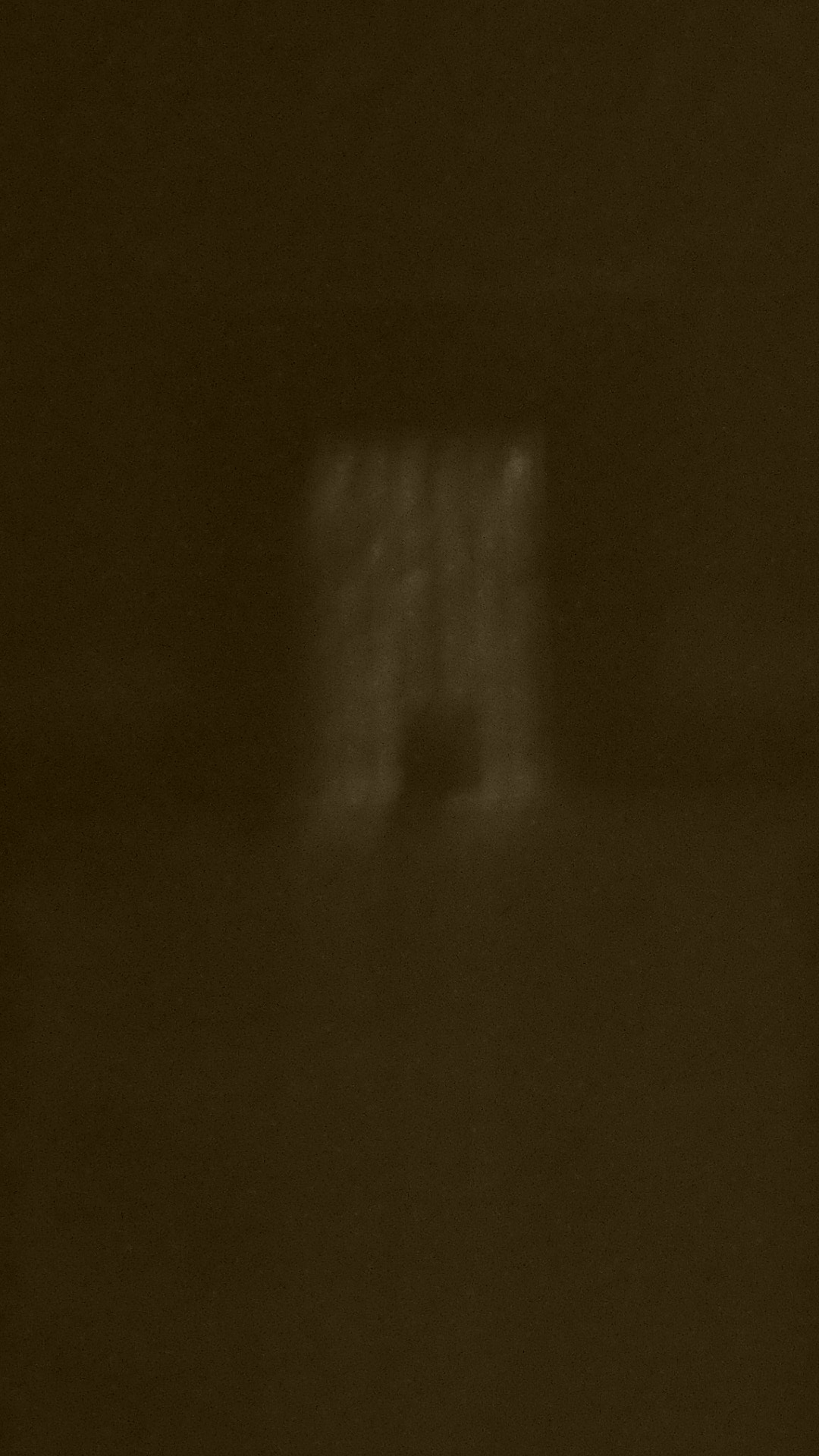This exceptionally blurry and dark photograph has a deep brown tint that varies slightly in intensity from top to bottom. The background features a primarily faded brown color that is darker at the top and lighter at the bottom. In the center of the image is a lighter brown vertical rectangle, which appears to have a square shape near its lower portion, possibly resembling a building with a door. The image suggests a bumpy texture around this central shape, implying some ground detail in front of the building. Additionally, there is a very faded white, square-like object visible in the distance. There is also a vague suggestion of a shadow, potentially of someone or something moving past the window-like structure, lending a ghostly, uncertain atmosphere to the scene.